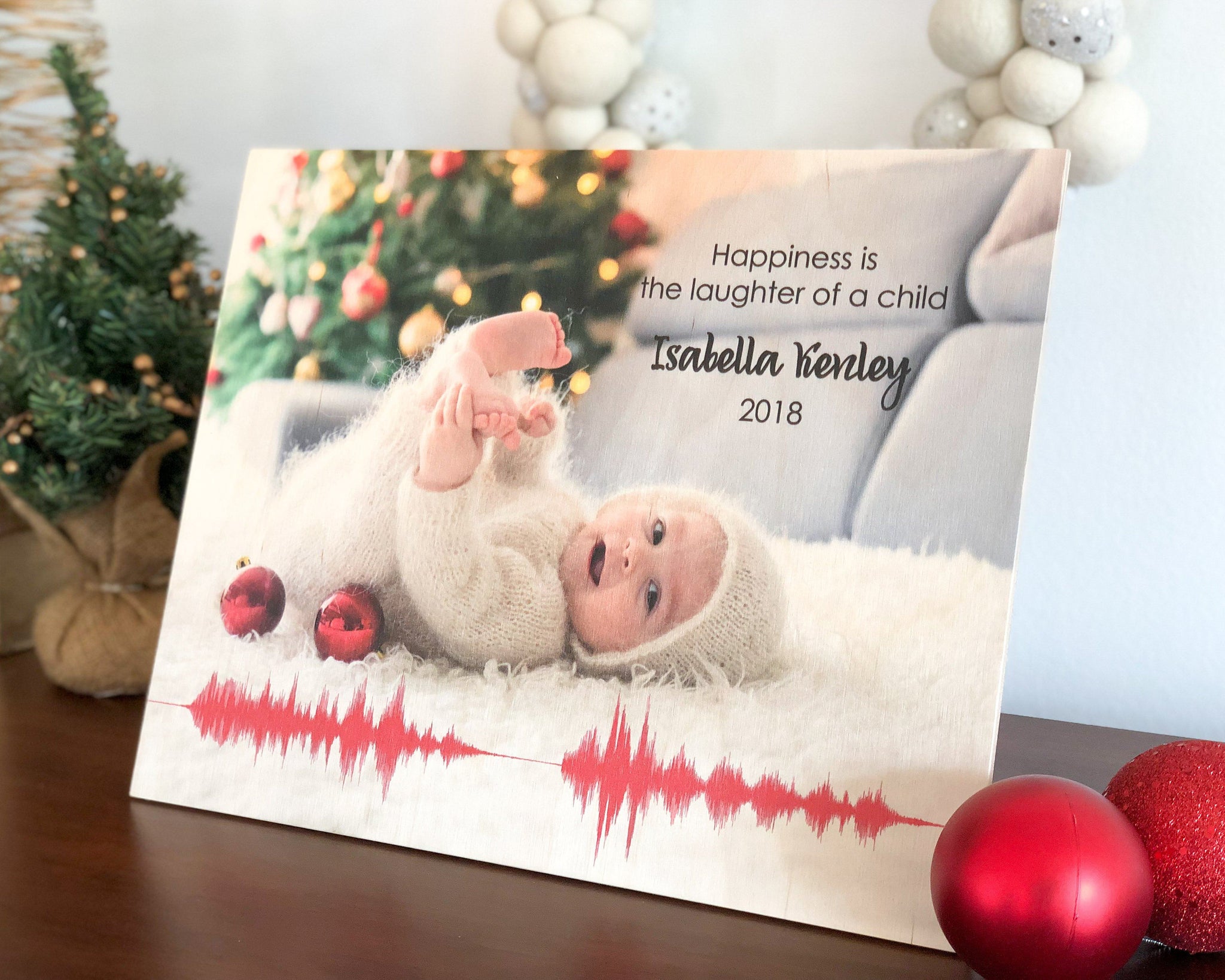The image is a color photograph of a Christmas-themed card resting on a dark brown wooden table. The card prominently features a white Caucasian baby laying happily on a fuzzy white rug, adorned in a matching fuzzy white onesie and hat, with its arms and legs stretched upwards. Surrounding the baby, towards the left are two round, shiny red Christmas ornaments, one smooth and one glittery, accompanied by a tiny artificial Christmas tree with green pines and little gold berries. Below the baby, there's a decorative red sound wave graphic symbolizing the child's laughter. The card bears the inscription "Happiness is the laughter of a child. Isabella Kenley, 2018" in the upper right-hand corner.